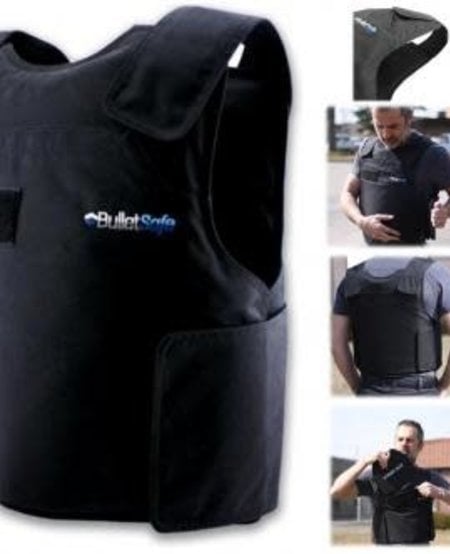The image is an advertisement for a bulletproof vest branded as "BulletSafe." Dominantly placed on the left two-thirds of the portrait image is a close-up of the black vest, emblazoned with the words "BulletSafe" — "Bullet" in white and "Safe" in blue — accompanied by a partially visible logo. The vest appears to wrap around the user, fastening with Velcro or clips at the shoulder and waist.

On the right one-third of the image, four smaller inset photos provide additional details. The top inset showcases the shoulder configuration of the vest, followed by an inset displaying a middle-aged white man, with short dark hair, putting on the vest from the front view. The third inset highlights the back view of the man wearing the vest over a shirt, while the final inset demonstrates the man adjusting or disassembling the vest, emphasizing its practicality and usage. The detailed imagery collectively portrays the vest's design, functionality, and ease of use, pointing towards its promotional intent, possibly for a catalog.